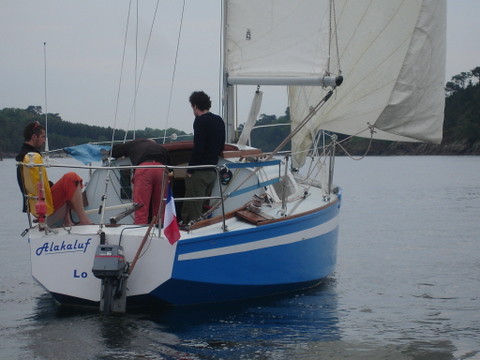The image portrays a detailed close-up of a sailboat named "Alakaloof," positioned on calm water, likely a lake or bay, with tree-covered hills visible in the background. The boat has a striking blue hull with a prominent white stripe and bears a French flag. It features an outboard motor at the back, where its name is inscribed along with the partial text "L-O."

Three men are aboard the sailboat. One man, seated on the left side with a life jacket on and a towel over his legs, wears a black shirt and long orange shorts, accessorized with sunglasses. Another man, positioned in the center, is bending over, possibly inspecting or adjusting something inside the cabin; he is dressed in a black shirt and green pants. The third man, also in a black shirt but with brownish pants, stands at the back, looking attentively at the central figure. The water around the boat appears tranquil, with no noticeable movement, implying that the sailboat is stationary.